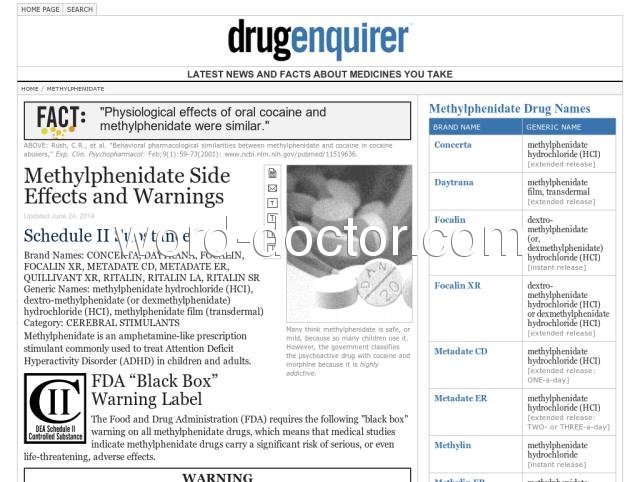This image features a webpage from Drug Inquirer, a website dedicated to the latest news and facts about medications. At the top left corner, two icons are visible: one for the homepage and another for the search function. Below these, the website's name is prominently displayed with "Drug" in black text and "Inquirer" in blue. The subtitle reads, "Latest news and facts about medicines you take."

Below the website's title, a headline in quotation marks announces the latest article: "Psychological effects of oral cocaine and methylphenidate or similar." To the right of this headline, the category is labeled “Methylphenidate Drug Names.”

The page then lists methylphenidate drug names, divided into generic and brand names. Although the very last name in the list is partially cut off, a total of eight names are mentioned, with generic names displayed in black text on the right side.

To the left, a section delves into side effects and warnings, starting with a detailed paragraph. This is followed by a notation referencing the "FDA" and a "black box warning label," accompanied by a couple of cautionary sentences. Positioned prominently at the bottom of this section is the word "Warning" in black text, enclosed in a rectangular border.

At the center of the image, a black-and-white photograph of pills is displayed, featuring a brief description beneath it in small gray text. The entire webpage is set against a clean, white background, providing a crisp and professional appearance.